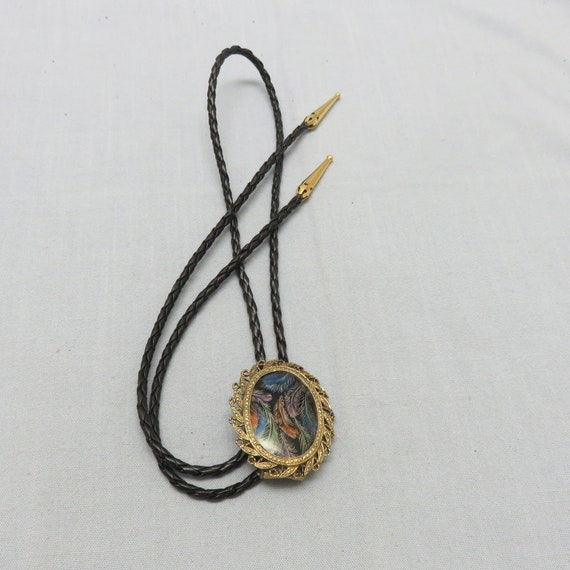This image features a decorative pendant reminiscent of a bolo tie, set against a subtle grey background. The pendant itself is an ornate oval piece, encased in a bronze-colored frame that's intricately patterned to resemble curved leaves enveloping the centerpiece. Within this sophisticated frame, a striking piece of art depicts an array of colorful feathers—swirls of orange, pink, green, blue, and shaded brown, arranged harmoniously against a black backdrop.

The pendant is secured by a black braided leather cord, adding a touch of rustic elegance. Each end of the cord is adorned with detailed, gold cone-shaped tips, matching the frame’s coloration and adding a sense of cohesion to the design. The pendant, with its artful and vibrant feather motif, sits gracefully atop the surface, possibly a white countertop, with the cord's ends neatly folded to the side. This piece of jewelry exudes a unique charm, blending artistic design with a touch of nature, making it a beautiful accessory likely intended for adornment.